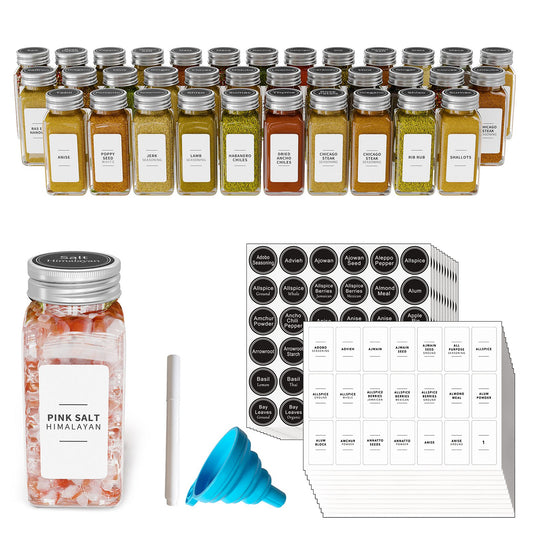This product photo showcases a sophisticated spice and herb collection, ideal for advertising. The image is divided into three clear quadrants. The upper portion displays approximately 30 clear glass bottles with silver caps, neatly arranged and pre-labeled with white rectangular labels, containing various spices and herbs. In the lower left corner, a single glass jar is prominently featured, labeled "Pink Salt Himalayan" with a black label on the top and a white label on the front. To the lower right, there's a chart that appears to provide a detailed list of the included herbs and spices, although the specific text is unreadable. A blue collapsible funnel is also visible in the foreground, adding a practical accessory to the ensemble. The background is stark white, emphasizing the product's clean and organized appearance. This image likely serves as part of a promotional campaign, highlighting the extensive and meticulously labeled spice system that includes both rectangular and circular labels, along with a marker for customization.